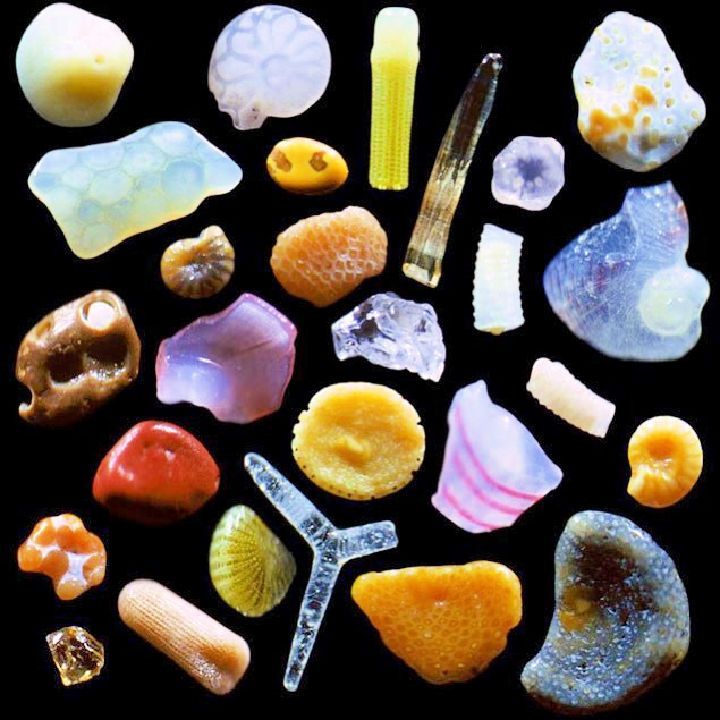In this photograph, a collection of approximately 30 distinct, natural objects is artfully displayed against a stark black background. Each item is clearly visible, positioned in a way that prevents overlapping, which allows the black background to prominently outline each object. The collection includes a diverse array of shapes, colors, and textures, reminiscent of what one might find during a scavenger hunt in a forest or on a beach. Among the assortment are round, cylindrical, and elongated stones with varying characteristics—some resemble seashells, diatoms, a miniature corn cob, and even a honeycomb structure. The stones and objects also showcase a vivid palette of colors, including yellow, orange, red, blue, pink, white, and brown. Highlighted pieces include a garnet-colored stone, an amethyst-hued gem, translucent crystals, and even objects that resemble a mollusk, a geode, and a loofah. Each object is unique, some appearing like phallic symbols or brown jelly candies, adding to the fascinating diversity captured in this detailed and visually striking image.